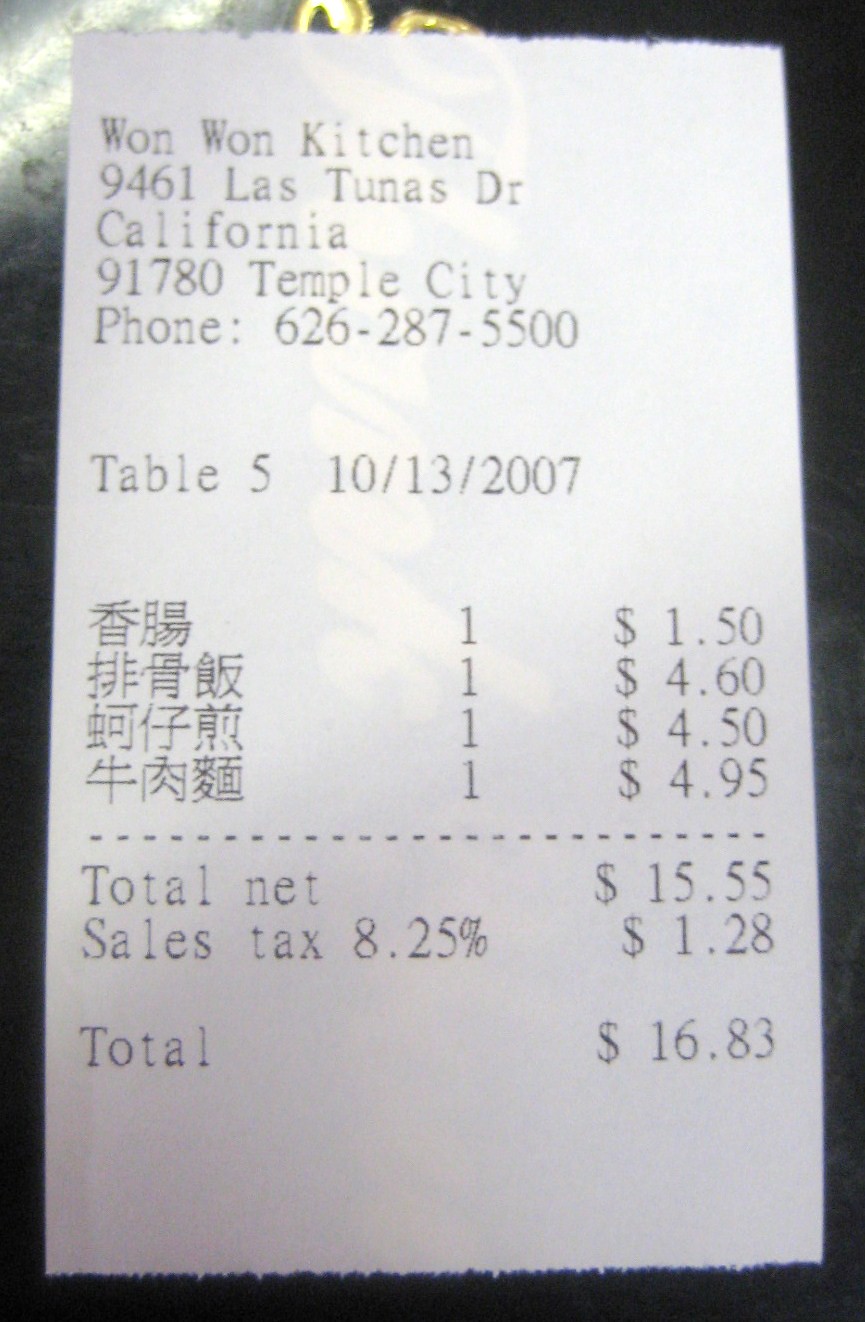This is a detailed photograph of a receipt from Wan Wan Kitchen, located at 9461 Las Tunas Drive, Temple City, California, 91780. The restaurant's phone number is 626-287-5500. The receipt is dated 10-13-2007 and is for table 5. The items ordered are listed in Chinese, with individual prices of $1.50, $4.60, $4.50, and $4.95, respectively. The subtotal amounts to $15.55. With an added sales tax of 8.25%, equating to $1.28, the total amount due is $16.83. The receipt appears to be placed on a black surface with faint gold writing partially obscured beneath it.